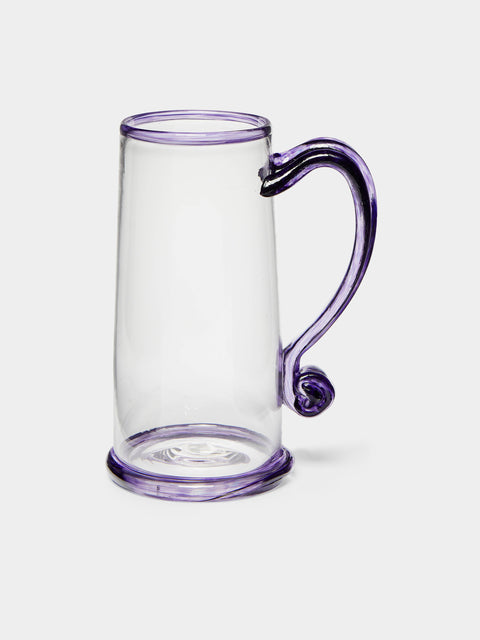This photograph features a distinctive clear glass mug set against a solid white background, likely taken in a photography studio for promotional purposes. The mug stands approximately eight to nine inches tall, with its clear, see-through glass slightly off-centered in the image. Both the top rim and the bottom base of the mug are accentuated by a thicker, transparent purple band, adding an elegant contrast to the otherwise simple design. The handle of the mug, positioned to the right, is an ornate, C-shaped structure that curves and coils akin to a decorative door handle, potentially forming a heart shape. The handle, also a transparent purple, adds a sophisticated and artistic flair to the overall minimalist yet fashionable aesthetic of the glass mug.